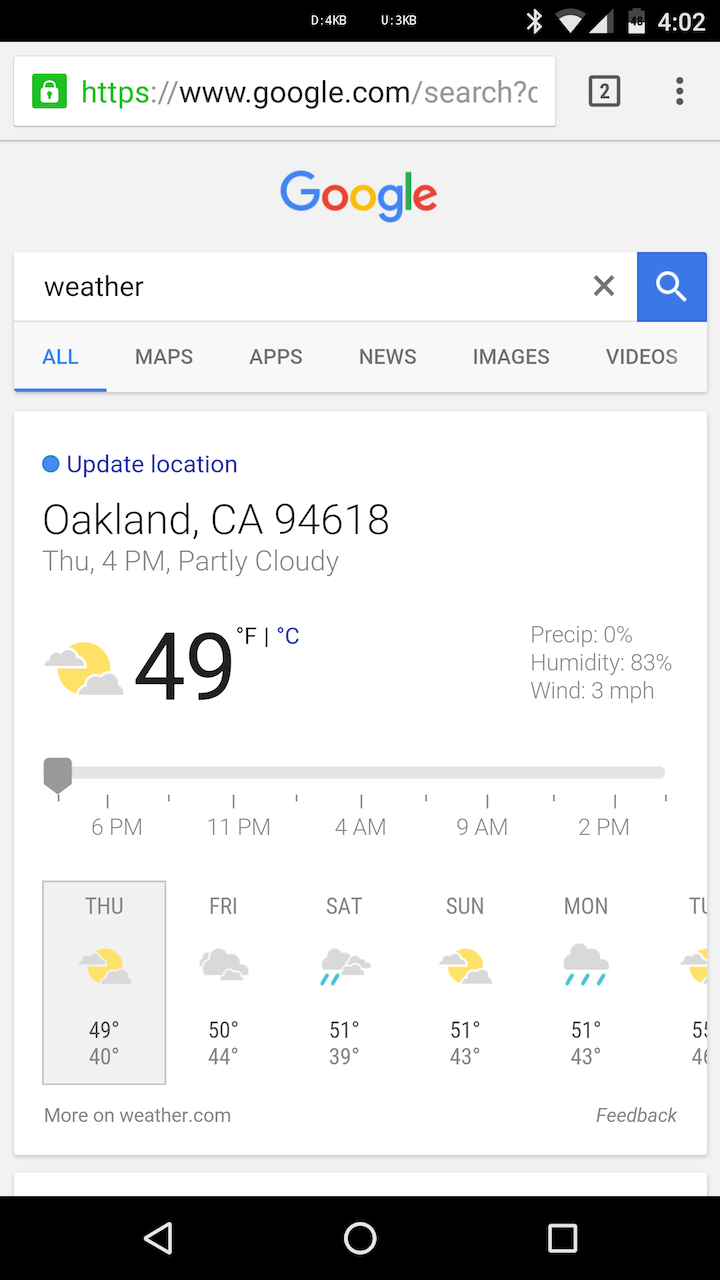This cell phone screenshot captures a detailed and organized display starting with the status bar at the top. On the right-hand side of this bar, the current time is shown, adjacent to a half-full battery icon, a three-quarters full signal bar, and a Bluetooth icon. There is also some faded, unreadable text or numbers in the center of the status bar.

Directly below the status bar, a search bar labeled with "https://" and "google.com" is visible, secured by a lock icon inside a green box to the left. The word "Google" is centrally placed within the search bar, exhibiting its traditional multicolored lettering. Inside the search bar is the query "weather," accompanied by an "X" icon on the left and a magnifying glass icon on the right.

Beneath the search bar, there are tabs labeled "All," "Maps," "Apps," "News," "Images," and "Videos," with "All" highlighted and underscored. The display centers around the weather information for Oakland, California, providing the current temperature of 49 degrees Fahrenheit. Additionally, it notes that it is Thursday and forecasts a low of 40 degrees for that day.